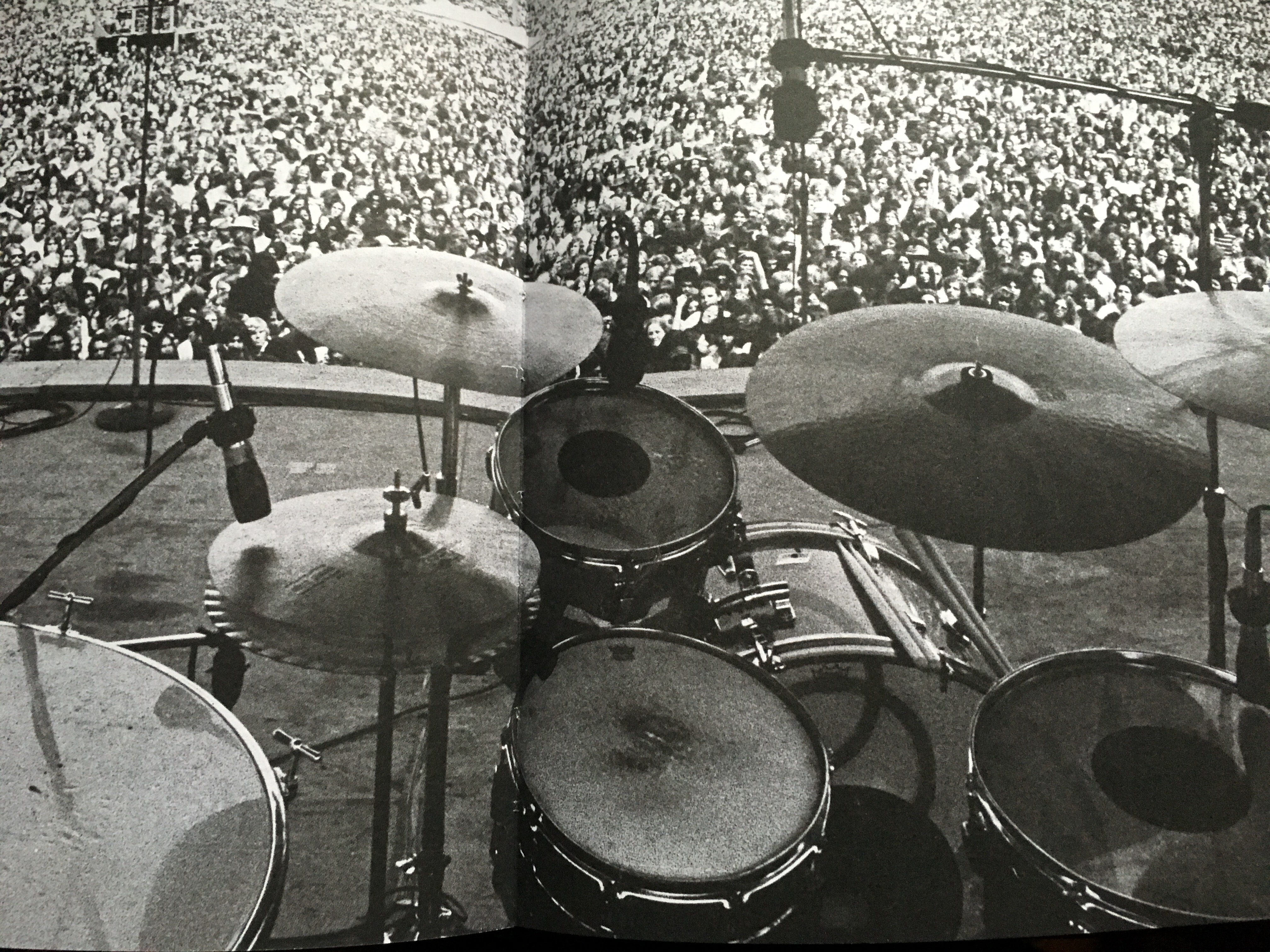In this close-up, black-and-white photograph, a detailed view of a drum set is captured on a stage before a massive, indistinct crowd. The drum set prominently features four cymbals, a bass drum at the center, a snare drum at the bottom, and two tom drums on either side. A hi-hat and multiple microphones are positioned around the drum set, suggesting it is set up for a live performance. The stage is devoid of people, emphasizing the equipment and the large audience in the background, which occupies the remainder of the image. The crowd appears as a blurred mass, making individual details undistinguishable. The black-and-white filter and overall composition suggest it might be an iconic concert event, possibly from an era like the 60s through the 90s, adding a historical or monumental significance to the scene.